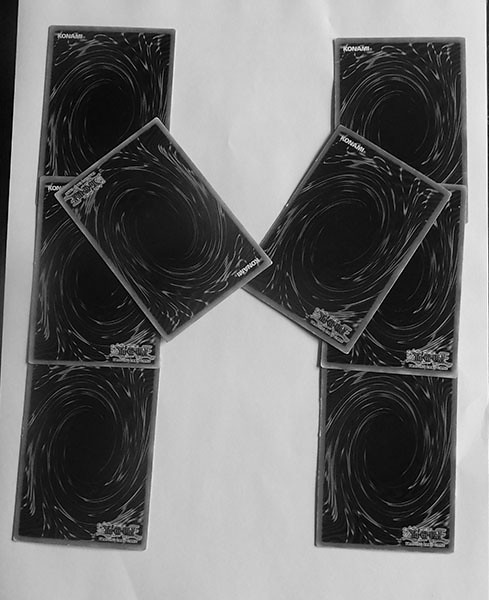The image showcases a collection of eight Yu-Gi-Oh! cards, identifiable by the text "Kanami" in the top left and additional text at the bottom right, likely indicating "Yu-Gi-Oh!". The cards feature a distinctive black and gray swirl pattern, resembling a portal or black hole. They are arranged on a white surface, possibly a blank piece of paper, in two neat columns of three cards each. Over each column, one additional card is positioned diagonally, almost forming the shape of an “M.” The organized yet dynamic layout highlights the intricate design of the cards against the contrasting white background.